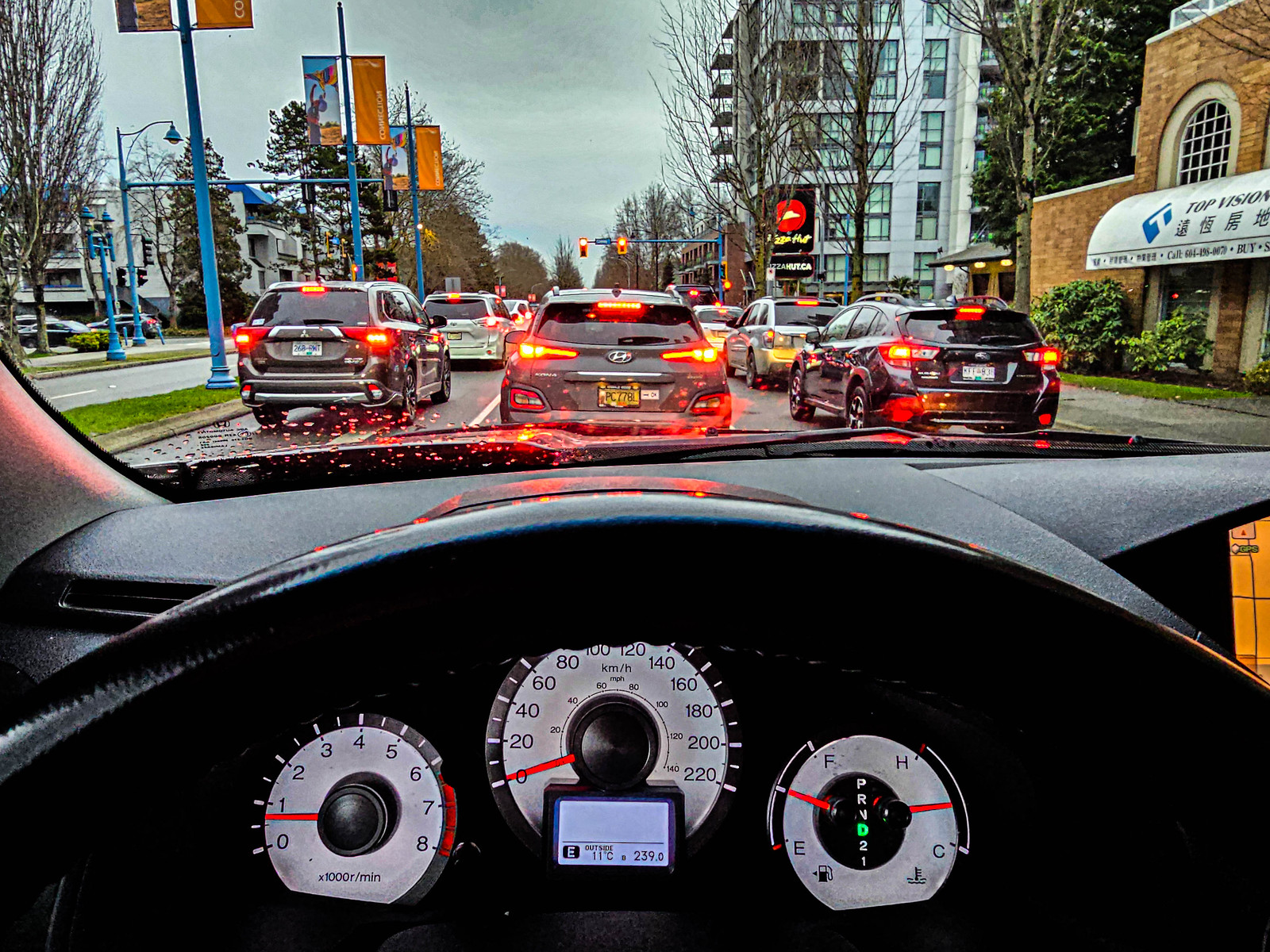The image, taken from within a car, captures the view from the driver's perspective. The foreground prominently features the car's black dashboard, showcasing various elements like the gear shifter, fuel gauge, and speedometer. Through the windshield, the scene transitions to the exterior, where a cloudy, gray sky looms overhead.

Directly ahead, three lanes of traffic are visible, populated with several cars. To the right, a series of large office buildings stand tall, accompanied by trees barren of foliage, revealing only their trunks, branches, and twigs. On the left side, a grassy area is interspersed with blue poles, topped with flags or banners fluttering in the wind. Beyond this, another lane of highway accommodates traffic moving in the opposite direction. Further left, another grassy stretch features similar blue poles, but these are equipped with streetlights.

Additionally, a road branches off to the side, where more cars can be seen navigating their respective paths. The overall composition of the image provides a detailed glimpse into the urban environment and the dynamics of the traffic situation.